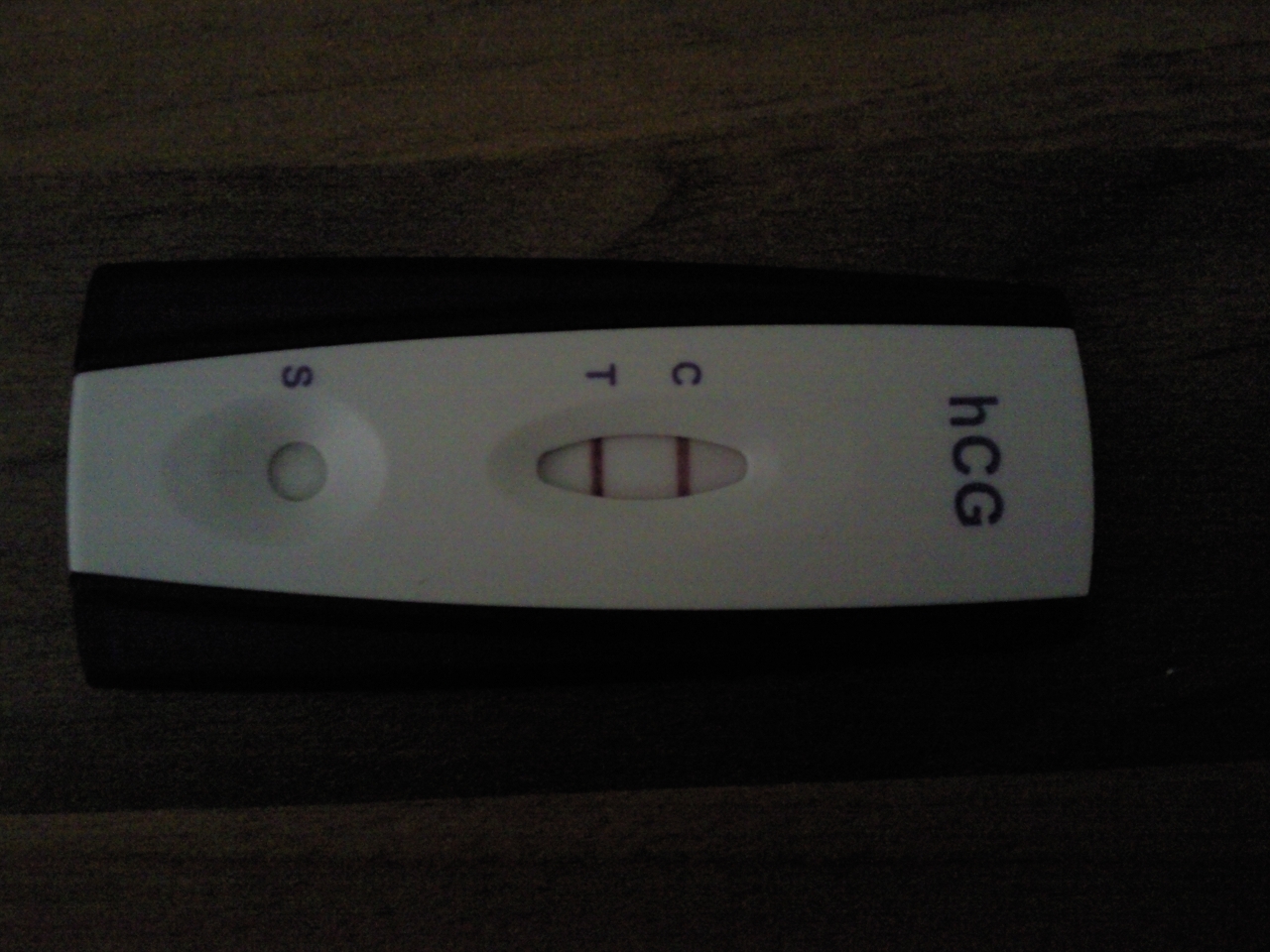In this image, a wooden tabletop serves as the backdrop, emphasizing the central subject: a pregnancy test. The test is rectangular with gently curved edges, designed for both functionality and comfort. A prominent white strip spans from the middle left side to the far right end of the device, gradually widening as it extends. On the left segment of this white strip, there is the letter "S," situated just above a circular indentation.

To the right of the indentation, the letters "T" and "C" are clearly marked. Directly below these letters lies a white oval slot, where two vertical red lines are visible, indicating the test results. Finally, at the extreme right end of the white area, small lowercase "h" and uppercase "CG" are printed, signifying the human chorionic gonadotropin hormone often tested for in pregnancy detection. The detailed design and clear markings make this pregnancy test both user-friendly and precise.